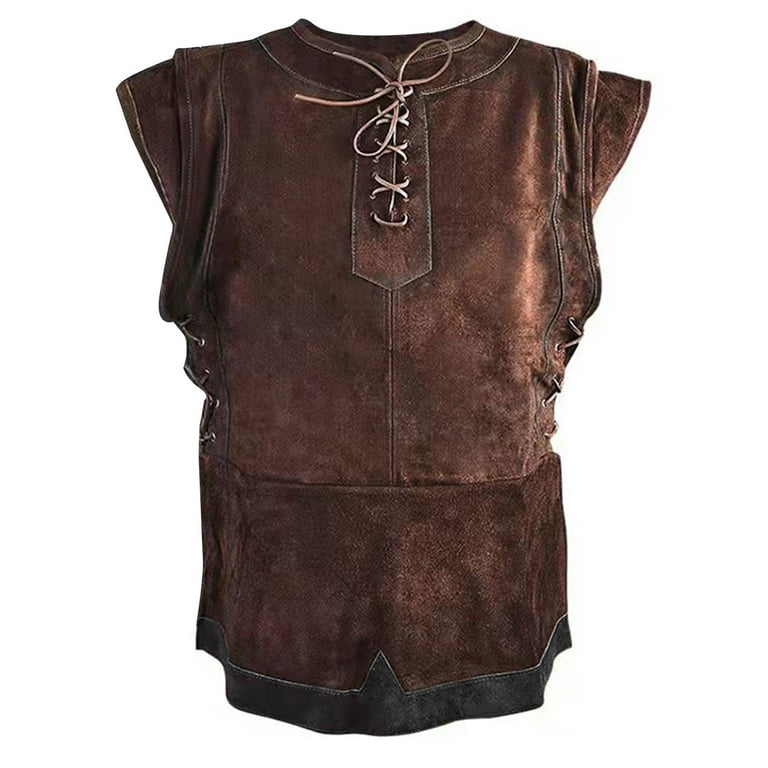This color photograph captures a detailed view of a vintage costume, set against a plain white background, exemplifying photographic representational realism in a portrait orientation. The subject is a dark brown leather tunic, almost suede in appearance, with unique characteristics. It features a typical crew cut collar with an opening at the front, threaded with a leather lace that ties into a bow, securing the neckline. The tunic has short cap sleeves and additional lacing on both sides under the armpits, allowing for adjustable tightness. The garment is unusually long, extending into a peplum-style skirt that gives the lower portion a somewhat skirt-like appearance. The hem at the bottom is crafted from a black leather piece, pointed at the center, adding a distinctive finish to the overall design.